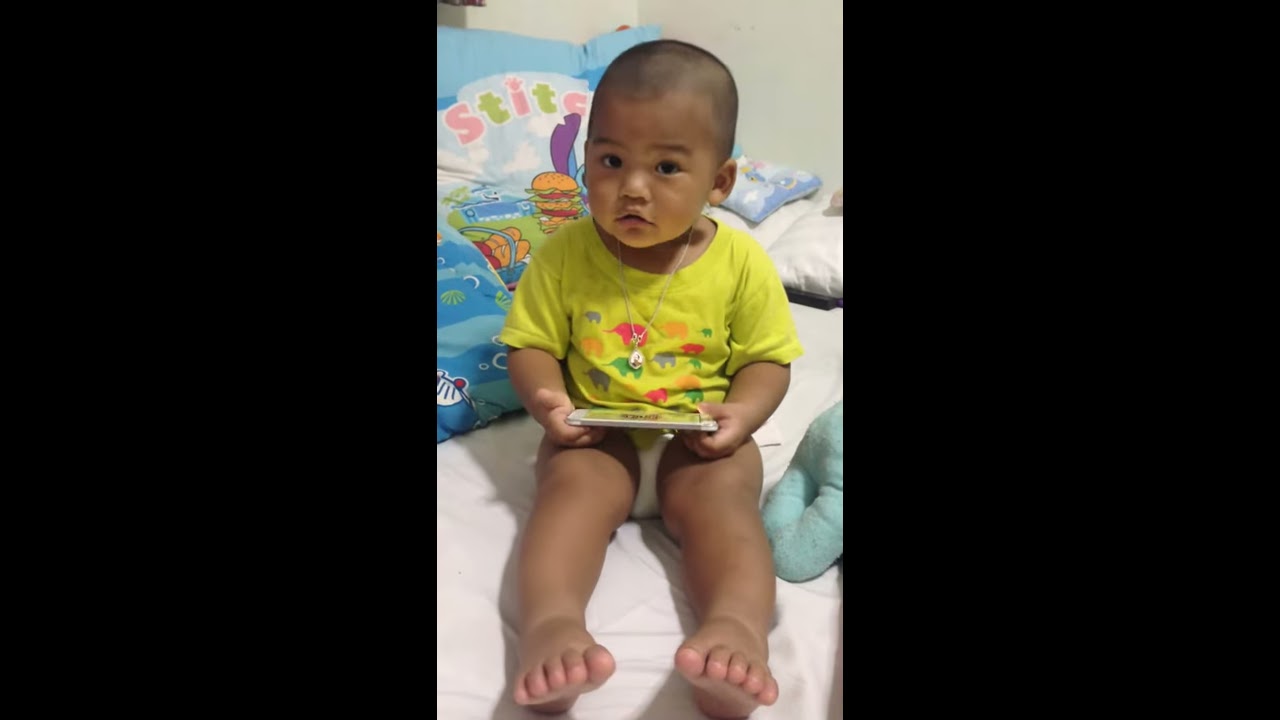In this image, a young child of around one year old is sitting on a white bedspread, surrounded by various pillows. The child has a darker complexion, dark hair, and dark eyes. They are dressed in a yellow shirt adorned with colorful elephants—pink, light blue, green, and orange—and a white diaper. Around their neck, they wear a necklace with a notable white base. The child is holding an object in their lap, which appears to be either a children's book or a tablet.

The scene is detailed with the child sitting upright, legs extended forward, showcasing their little toes in the foreground. Behind them, several pillows are arranged, including one featuring cartoonish decorations with a hamburger and some lettering beginning with "S-T-I-T," possibly part of the word "Stitch" with an image of Stitch holding a hamburger partially visible. A blue pillow is also noticeable on the right side of the child. The child's expression is neutral as they gaze into the camera.

The setting appears to be in the corner of a room, with a white wall visible right behind the child's head, adding a dimensional backdrop to the cozy and intimate scene. The photograph is displayed in the central panel of a triptych layout, with two blank black panels flanking either side.